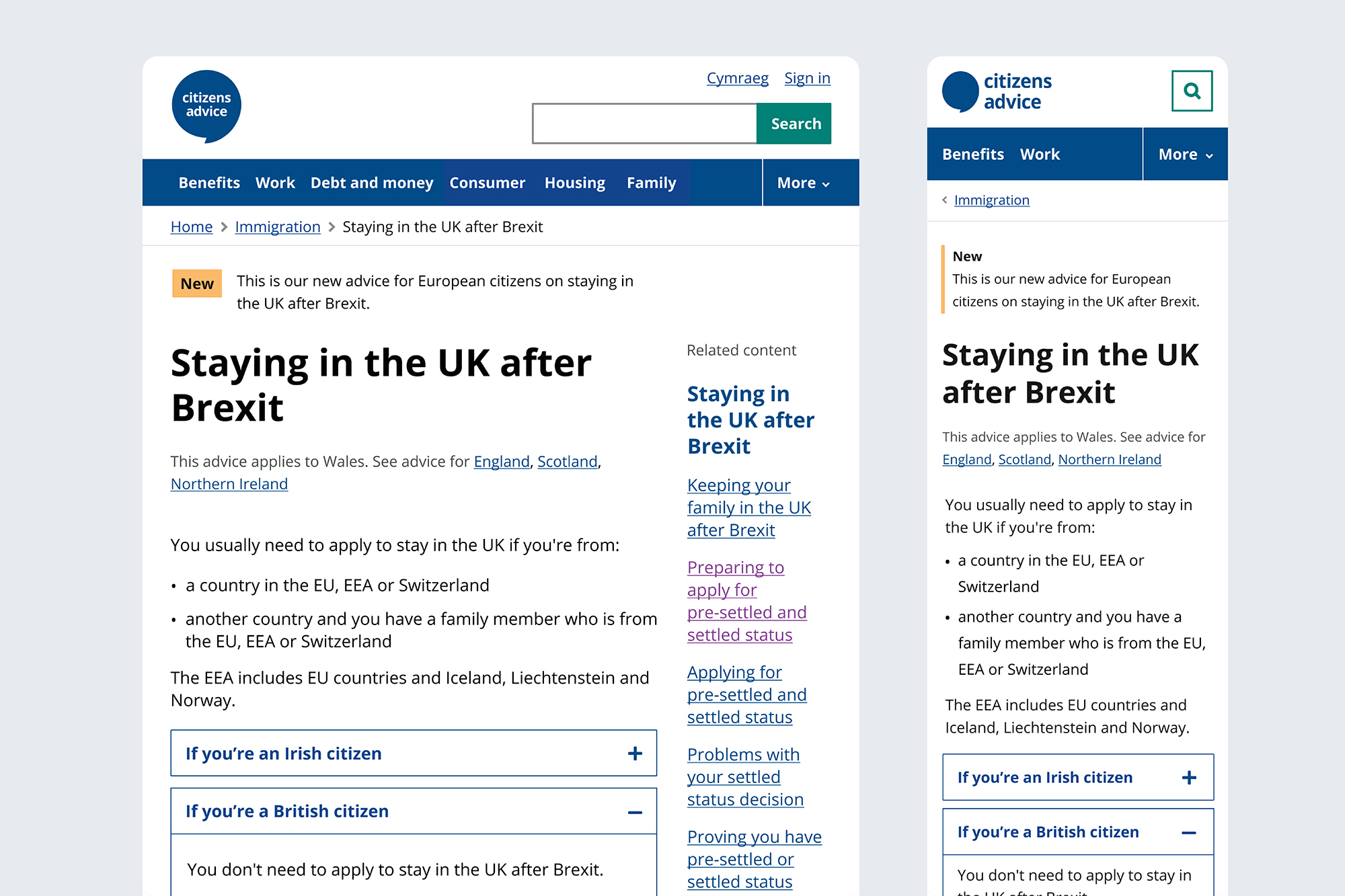The image displays the Citizens Advice website interface. In the top left corner, there is a white "Citizens Advice" logo set against a dark blue circular background. Adjacent to the logo, towards the right, is a rectangular search bar, featuring the word "Search" on a green background. Above this search bar, there is a blue sign-in button.

To the right of this initial interface, the image showcases a mobile version of the same website, which mirrors the desktop layout: it has the Citizens Advice logo and name on the top left, along with a search bar situated on the top right.

On the desktop view, spanning across the top middle left area, are several navigational categories listed horizontally. These categories are: Benefits, Work, Debt and Money, Consumer, Housing, Family, and More. The "More" category includes a downward arrow to indicate a dropdown menu.

Beneath these navigational categories, in the middle of the left section, there is a message that reads "Staying in the UK after Brexit. This advice applies to Wales." This is followed by a prompt to "See advice for England, Scotland, Northern Ireland," with the names of these countries in light blue, underlined text, indicating that they are hyperlinks.